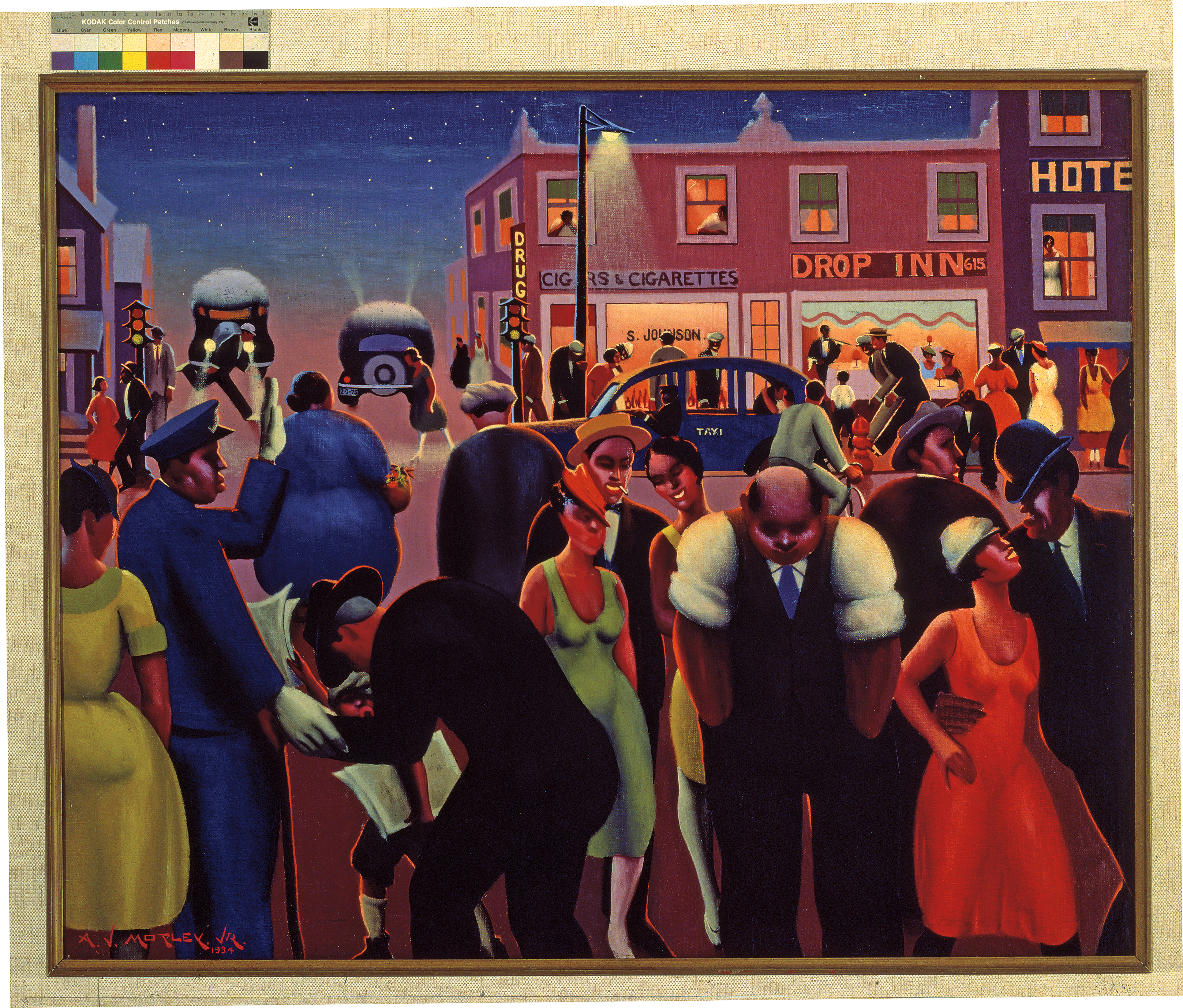The image depicts an Art Deco style painting of a bustling nighttime city scene. The painting, framed in dark wood, features a dark blue sky streaked with white stars. The cityscape below is adorned with angular buildings, including a suburban house with a traffic light on the left and a downtown area on the right. The prominent red building in the center displays signs reading "Drugs, Cigars, Cigarettes, S. Johnson, Drop-In, 615,” while a taller purple building further to the right has a "Hotel" sign. The streets are alive with activity, featuring cars driving on a snowy pink surface and a blue taxi in front of the hotel. Numerous black individuals, smartly dressed in suits and dresses, fill the sidewalks and streets, suggesting they are either heading out or returning from a night on the town. Among the crowd, a policeman in a blue uniform with white gloves directs traffic, and there's a man walking with a cane, indicated to be receiving assistance from the officer. In the mix, a little boy appears to be selling newspapers. The painting's bottom left corner holds an illegible red signature. Accompanying the painting in the photograph is a beige woven surface and a Kodak Color Control Patches card, hinting at the photographic documentation process.